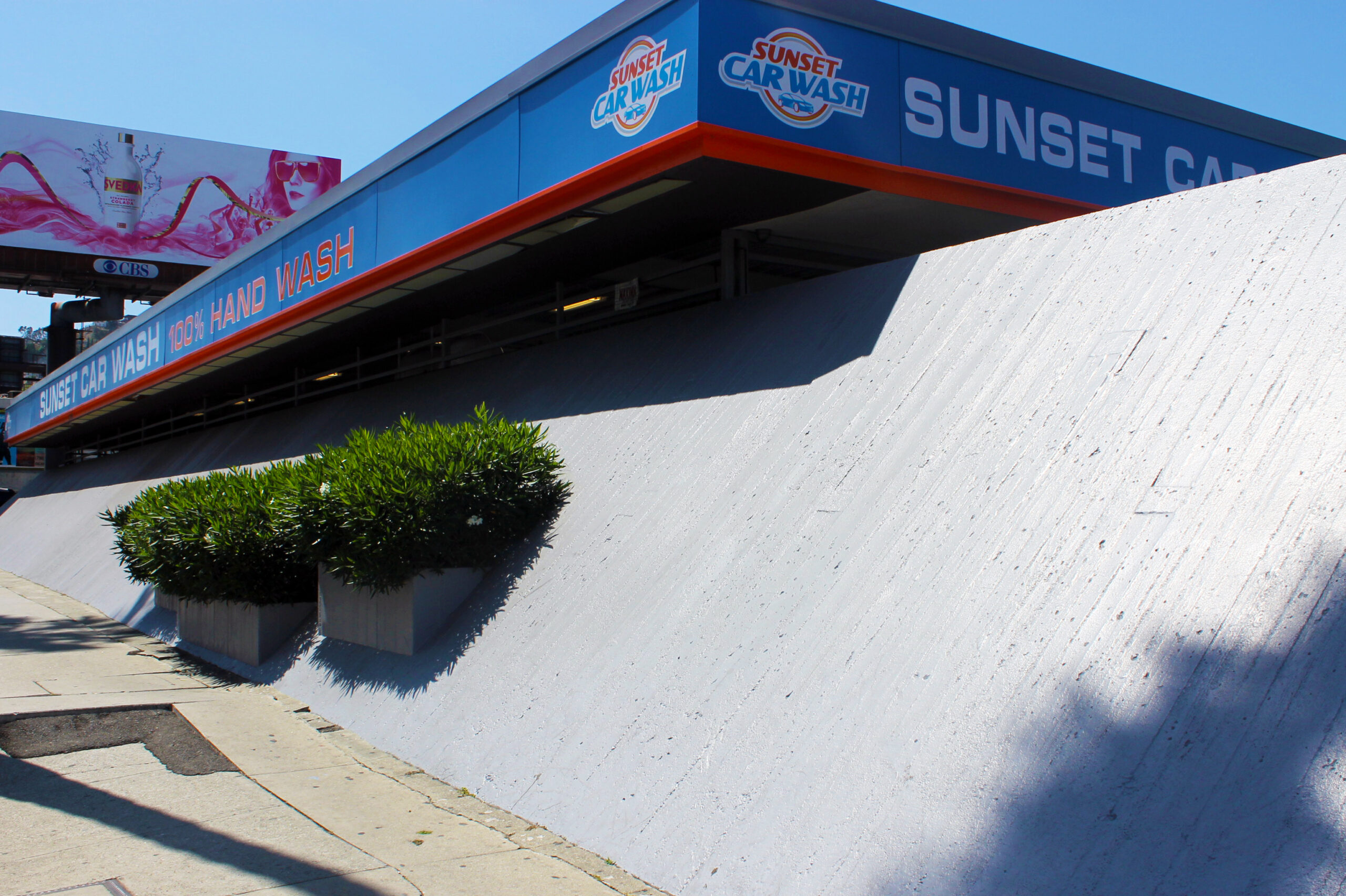The image depicts an outdoor setting featuring a distinctive car wash structure. Central to the scene is a concrete barrier that rises at a steep angle, appearing white or silverish. This barrier, dotted with square outcrops containing vibrant green shrubs, creates a dynamic foreground. Hovering above the barrier is a striking rooftop of the car wash, adorned in blue and casting a considerable shadow over the concrete below. Prominently displayed on the rooftop is the "Sunset Car Wash" logo, with "Sunset" in red and "Car Wash" in blue. This text is repeated in white alongside the phrase "100% hand wash" in red, all forming part of the establishment’s branding. To the far left of the scene, a billboard with a white background features an image of a woman, a bottle, pink ribbons, and flowers, hinting at a shampoo or conditioner advertisement. The entire scene is set against a clear blue sky, enhancing the vibrant details and colors of the car wash signage and the lush greenery.